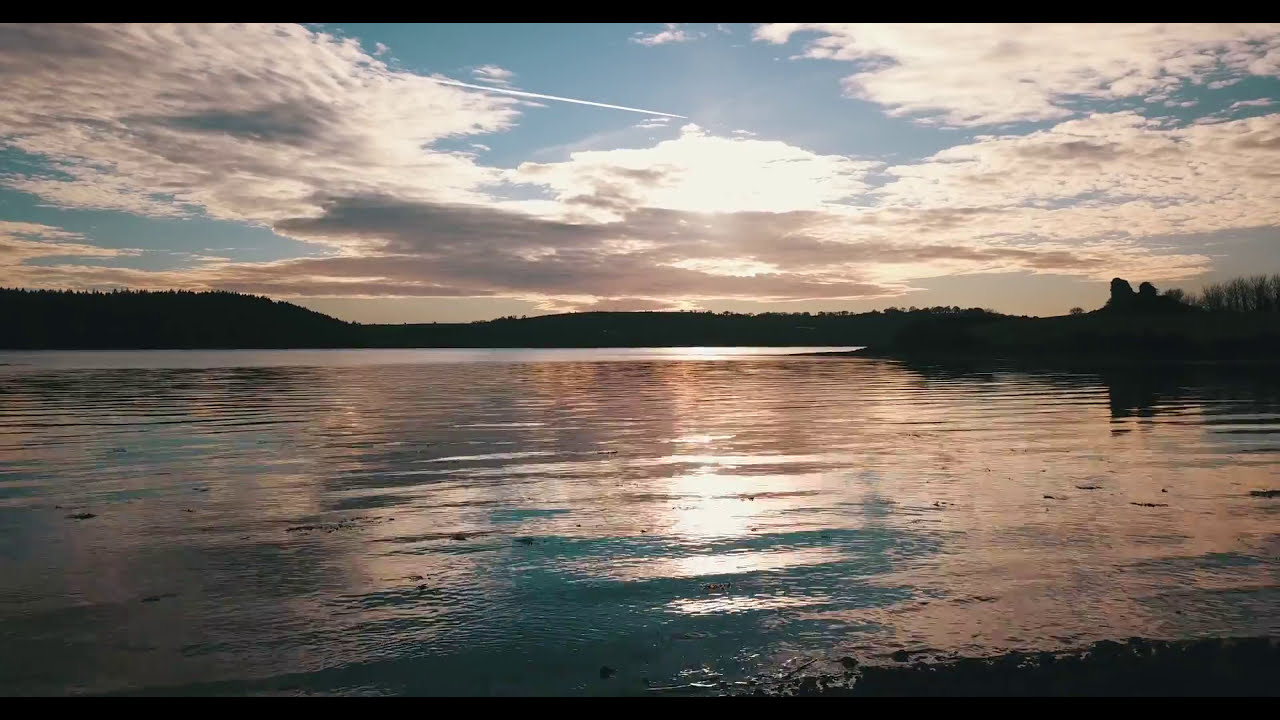This color photograph, oriented in landscape, captures a serene and expansive lake at sunset from the viewpoint of the lakeshore. The sun sits low in the sky, barely peeking through thick, dark clouds that allow golden sunbeams to stream through. The sky transitions from a lighter blue to dark hues, embodying the closing moments of daylight. Cirrus clouds mingle with grayer rain clouds on the horizon, intensifying the dramatic effect. The photographer's vantage point includes a slight shoreline visible in the bottom right corner, where ripples in the water suggest gentle movement. The lake beautifully mirrors the encircling trees and the dusky landscape, with a distant shoreline of hills and woods, casting dark reflections. The image emphasizes photographic representational realism, capturing the tranquil and picturesque atmosphere of a sunset over a secluded, wooded lake.